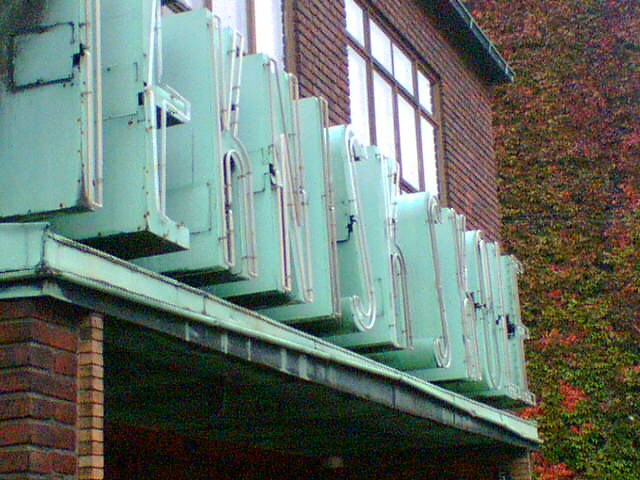In the image, a striking red brick building stands prominently. A column of exposed red bricks is visible on the bottom left side, adding texture to the facade. A horizontal green ledge extends across the building, resembling a garage entrance underneath. Above this green structure, block letters spell out what appears to be a name or sign in green with a white outline. Further up, the red bricks frame two windows, enhancing the building's rustic aesthetic. A black roof crowns the structure, contrasting sharply with the red bricks. To the right, vibrant greenery punctuated by pink flowers creates a picturesque foreground.